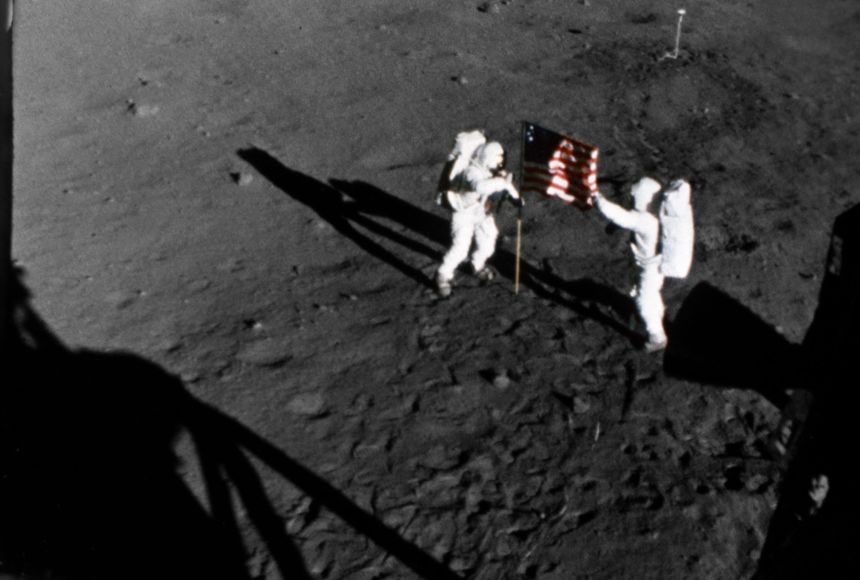This black and white photograph, taken from the Lunar Lander, captures a historic moment of the moon landing. Centered in the image, two astronauts in full white spacesuits with large white backpacks stand on either side of an unfurled American flag. The surface of the moon, depicted in a gray, pitted landscape with numerous craters, extends beneath them. The astronaut on the left grips the wooden flagpole, while the one on the right holds the flag's edge. Heavy black shadows, including those cast by the astronauts and the Lunar Lander, stretch across the moon's uneven terrain. The flag itself features the iconic red and white stripes with a navy blue canton adorned with stars. The shadow of the Lunar Lander is visible in the lower left corner of the image, emphasizing the scene's otherworldly setting.